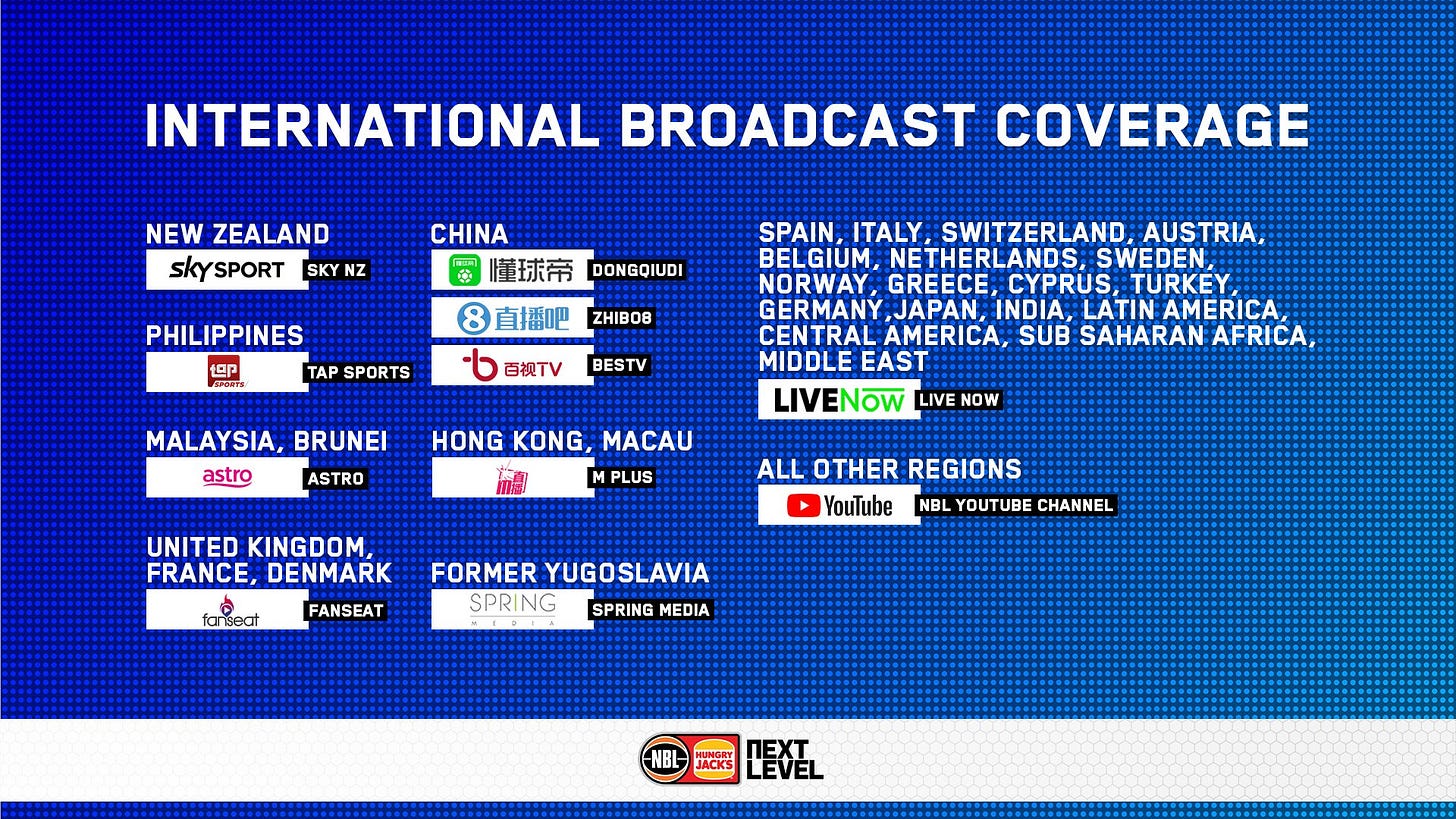The image resembles a screen from a sports broadcast, showcasing international coverage for an event. The blue background features lighter blue dots for texture, with larger white text in the center reading "International Broadcast Coverage." Below, three columns list various regions and their respective broadcasters. 

In the first column, New Zealand is covered by Sky Sport; the Philippines by Tap Sports; Malaysia and Brunei by Astro; followed by the United Kingdom, France, and Denmark, all covered by Fan Seat. 

The second column lists China with three distinct broadcasters: Dong Quidi, Zhi Bo, and BesTV. Hong Kong and Macau are covered by M+; and former Yugoslavia by Spring Media.

The third column is extensive, covering Spain, Italy, Switzerland, Austria, Belgium, Netherlands, Sweden, Norway, Greece, Cyprus, Turkey, Germany, Japan, India, Latin America, Central America, Sub-Saharan Africa, and the Middle East, all under the broadcaster Live Now. For all other regions, coverage is available on the NBL YouTube channel.

At the bottom, a white bar is prominently featured, centered with the text "Next Level" and flanked by the NBL logo on the left, displaying "NBL" within a circle and a logo reminiscent of the Hungry Jack's branding on the right.